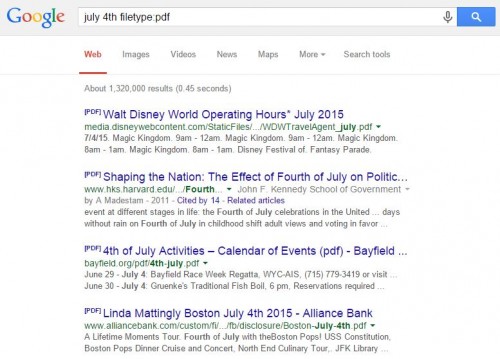Screenshot of a Google search results page. The page features a clean white background, with the familiar tan-colored top bar where "Google" is displayed in its iconic, multi-colored font in the left corner. On the right side of the top bar, a search magnifying glass icon is situated against a blue background, and immediately to its left is a microphone icon. The search query entered in the search bar reads: "July 4th file type: PDF."

Directly below the top bar, there are navigation tabs labeled "Web," "Images," "Videos," "News," "Maps," "More," and "Search tools." These tabs allow users to switch between different types of search results. Beneath this navigation, in the central area of the page, are the text results relevant to the search query. These include:

- "PDF Walt Disney World operating hours July 2015."
- "PDF Shaping the Nation: The Effect of 4th of July on Politics."
- "PDF 4th of July Activities Calendar of Events."
- "PDF Bayfield."
- "PDF Linda Mattingly Boston July 4th 2015 Alliance Bank."

The page layout aligns with Google's standard interface, presenting users with a clear and user-friendly way to navigate search results specific to PDF documents relating to July 4th.